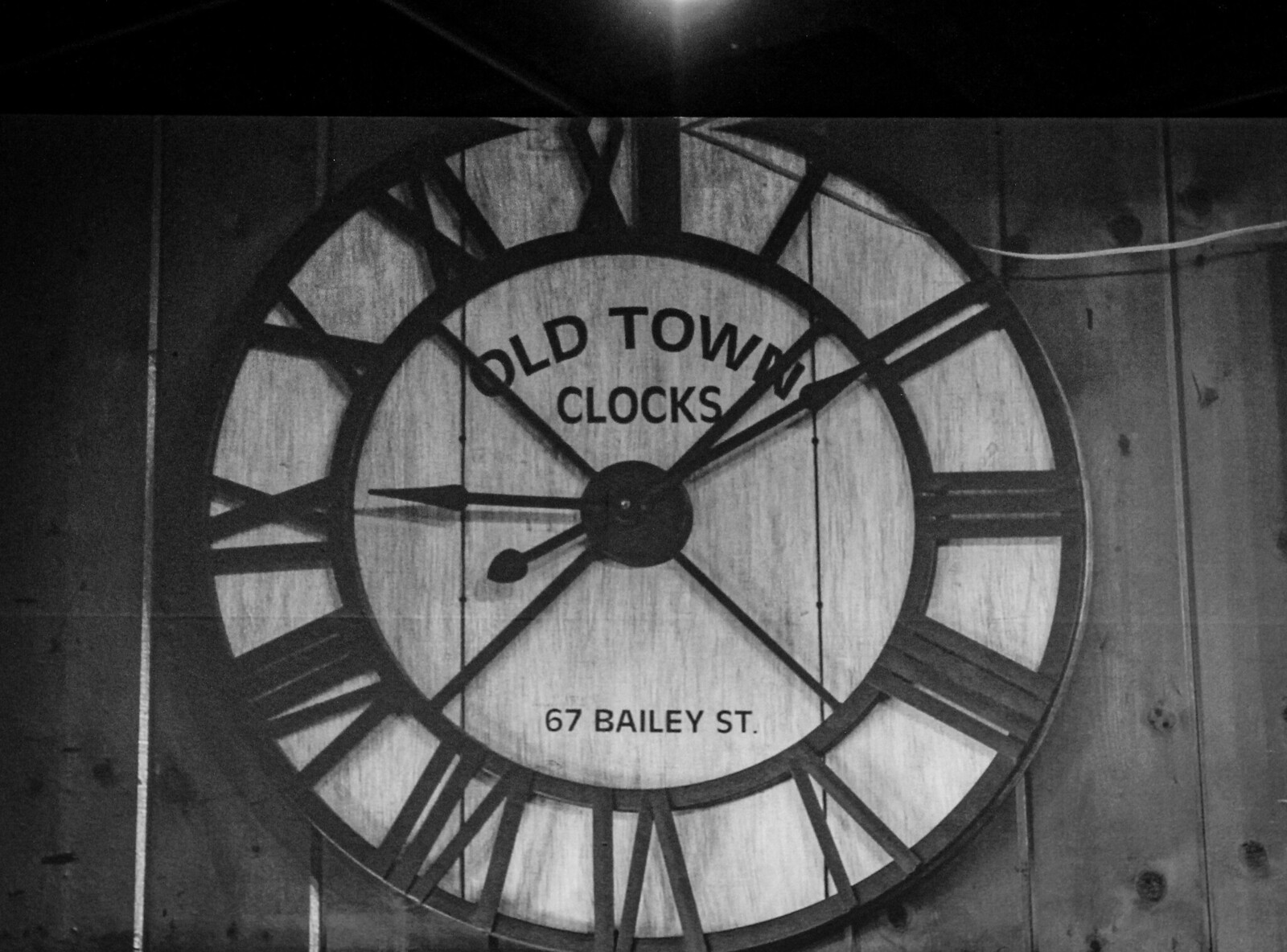This black and white photo captures a detailed, rustic scene featuring a large, circular clock mounted on a wall of weathered pine boards, which have turned a grayish color. The clock, which exudes an old-fashioned charm, has a black ring outer circle with a smaller inner circle inside it. Sandwiched between these circles are the hour markers in Roman numerals. The clock face prominently displays black lettering that reads "Old Town" with "Clocks" beneath it, followed by an address in gray letters, "67 Bailey Street." The current time shown by the clock is 9:10, with the hour hand at the nine o'clock position and the minute hand pointing to the two. There may also be a second hand positioned between the four and five. Adding to its rustic appearance, a wire drapes over the top of the clock, and it looks like there's a light source above, suggesting it might have been taken in low light conditions. Overall, this large metal clock stands out against the distressed wood backdrop, creating a nostalgic and timeless scene.